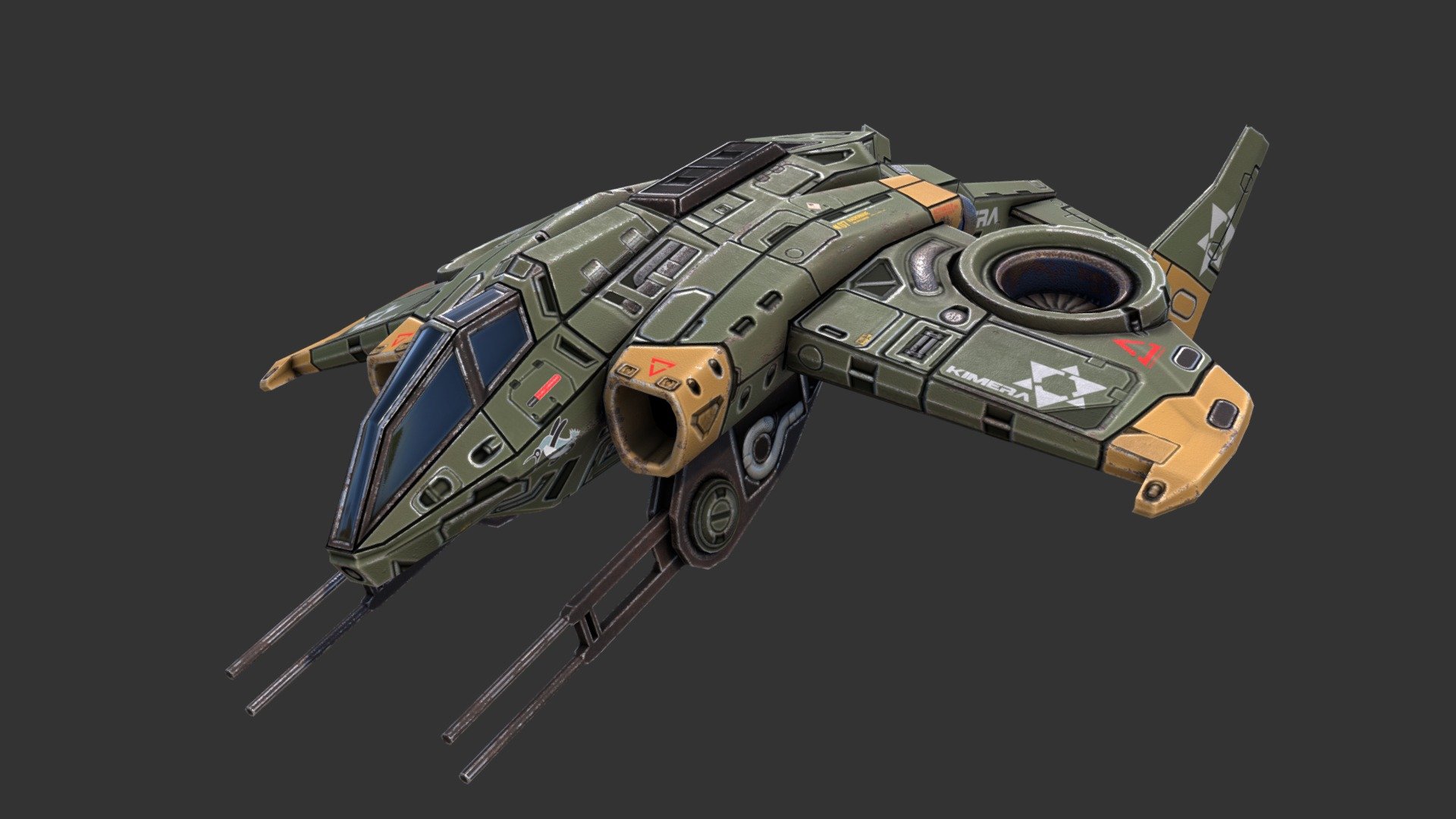The image displays a digitally created, futuristic aircraft that appears to be concept art or a 3D model, likely from a video game. The aircraft, a blend between a helicopter and a jet, is designed in a dark, navy green color with yellow-tinted wings and tips. Prominently, it features large, multi-angled turrets—one protruding from the bottom and another from the front. The guns are rustic and metallic, with prong-like points suggesting powerful shooting capabilities. The cockpit boasts a large, arched window with a noticeable blue hue. An eye-catching demonic star design adorns one of the wings, and next to it, the word "Chimera" is inscribed in white. Red accents are subtly interspersed across its metallic body. The craft is centered against a dark gray background, highlighting its intricate, futuristic details.